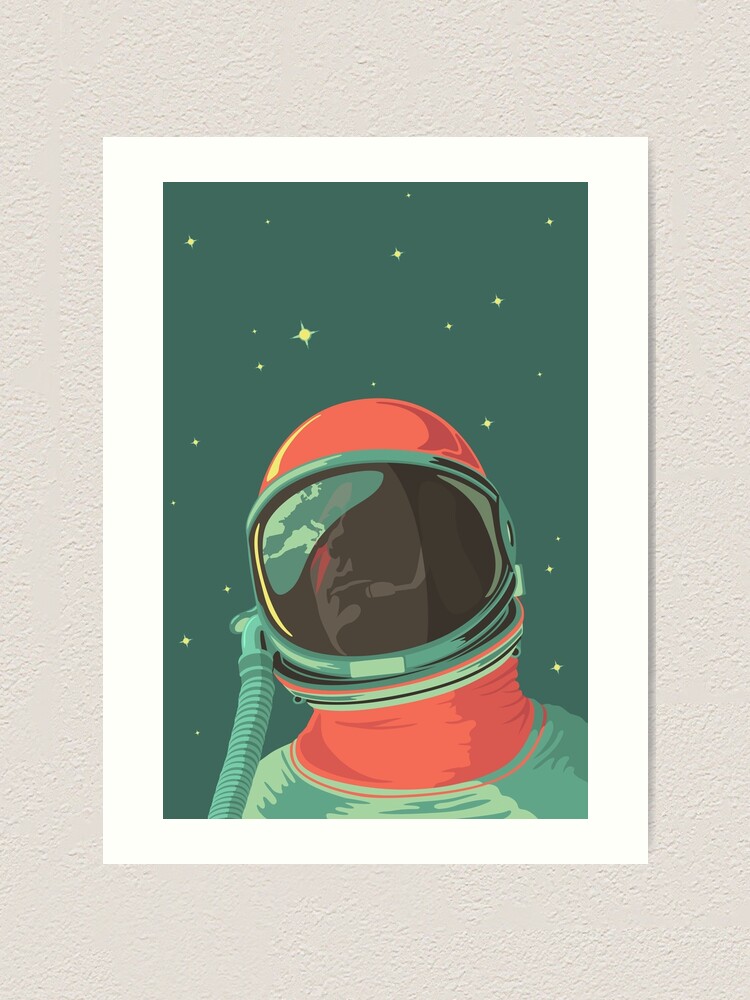This is a detailed illustration, presented on matte paper against a cream-colored textured wall, with a pure white border framing it. The primary subject is an astronaut depicted from the shoulders up, clad in a space suit. The helmet is a striking red or corally pink color, with a large visor that covers the entire face, providing a reflective view of the Earth or possibly clouds. There is a visible tube attached to the helmet, likely to supply oxygen. The rest of the suit incorporates light green, teal, or white hues. The background behind the astronaut is a deep green or turquoise space, dotted with various sizes of stars, setting an otherworldly scene. You can faintly discern the astronaut’s face and a small microphone in his helmet, adding a touch of realism to the graphic print. This piece would make a captivating addition to any wall, whether framed or unframed.